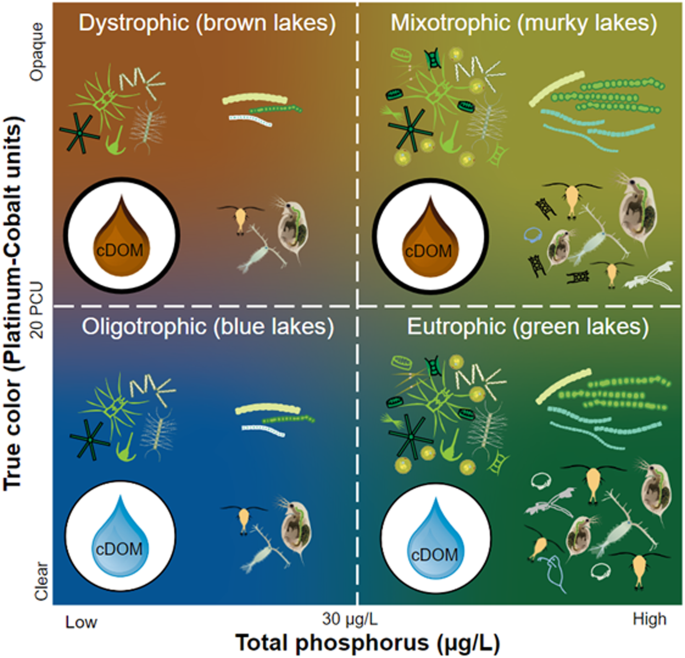This detailed illustration, likely from a textbook on lake ecology, is a square graph divided into four quadrants, each representing different lake types based on their color and nutrient content. The vertical axis is labeled 'True Color Platinum Cobalt Units,' ranging from clear at '0 PCU' at the bottom to opaque at '20 PCU' at the top. The horizontal axis is labeled 'Total Phosphorus, micrograms per liter,' spanning from low concentrations on the left to high concentrations up to '30 micrograms per liter' on the right.

Each quadrant is color-coded and labeled to depict specific lake types:
- **Upper Left (Dystrophic Brown Lakes):** Brown background, indicating high organic content and low phosphorus.
- **Upper Right (Mixotrophic Murky Lakes):** Murky background, showing a mix of moderate phosphorus and color.
- **Lower Left (Oligotrophic Blue Lakes):** Blue background, representing low levels of nutrients and clear water.
- **Lower Right (Eutrophic Green Lakes):** Green background, indicative of high nutrient levels and potential algal blooms.

The background colors in each quadrant blend into one another, creating a gradient effect. Each section also features illustrations of the microscopic life forms typical for each lake type, emphasizing the ecological diversity and chemical composition across different lake environments.